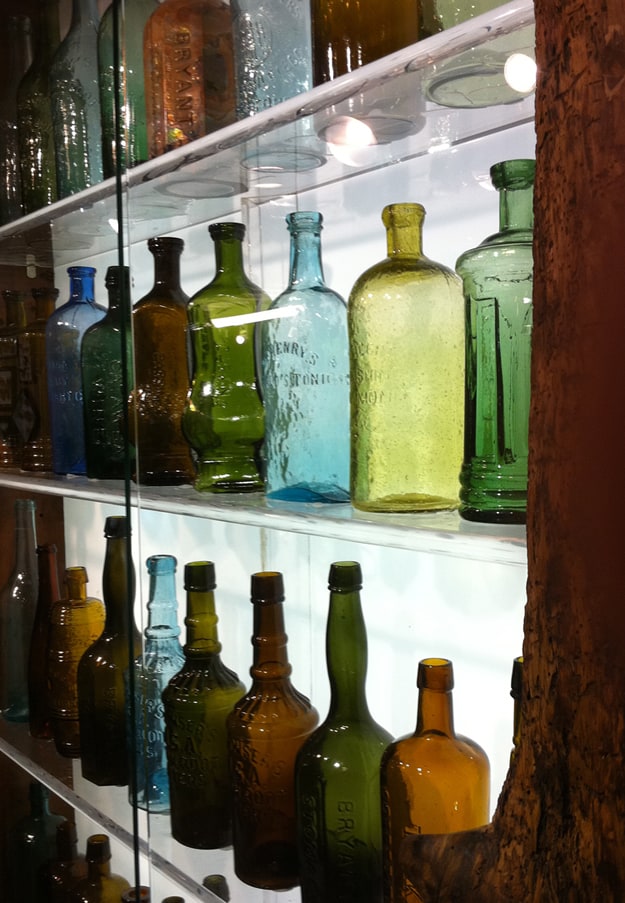The image is a detailed photograph of a glass cabinet packed with an array of elaborate, antique glass bottles in various colors, including green, blue, yellow, orange, dark brown, and bronze. These bottles, some with intricate necks and unique lips, are displayed across multiple glass shelves—two are fully visible, a third is partially visible at the bottom, and the top shelf shows the bases of more bottles through the glass. The shelves are backlit against a white wall which illuminates the bottles, creating a striking effect. The cabinet is behind a glass panel, featuring a brown wooden post that spans the entire right side of the image, likely part of the shelving structure itself. The glass doors reflect the light, adding depth to the scene.